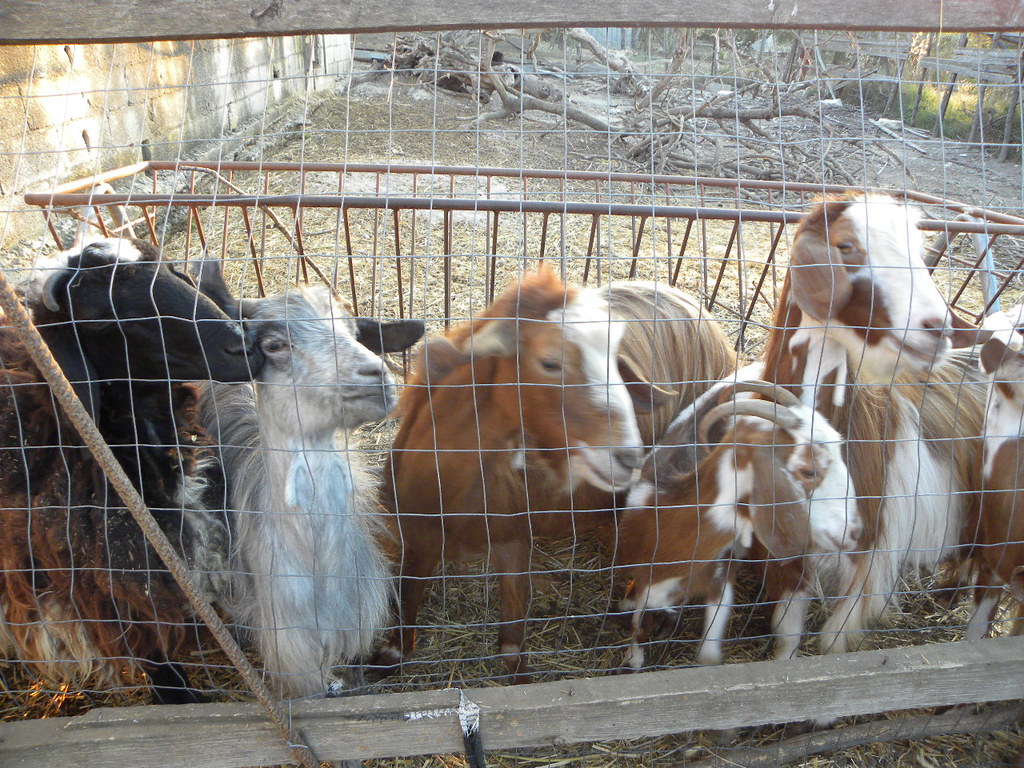The image features a pen at a zoo during the daytime, encased by a wooden-framed fence topped with chicken wire. Directly at the forefront, but behind the chicken wire barrier, there are six visible goats, ranging in color: a black goat, a white goat, a brown goat, a brown and white goat, another brown and white goat, and part of another goat at the edge. The goat at the bottom right stands out with large, round brown horns. The animals appear to be looking towards the camera, occupying most of the image. The ground within the pen is a mix of dry hay and dirt, with minimal foliage. In the background, against a cinder block wall marked by varying shades of discolored tan paint, lies a large fallen tree with bare, broken branches. Some green foliage can be seen further in the background, providing a contrast to the otherwise dry environment. Overall, the scene suggests a somewhat crowded and dirty enclosure.